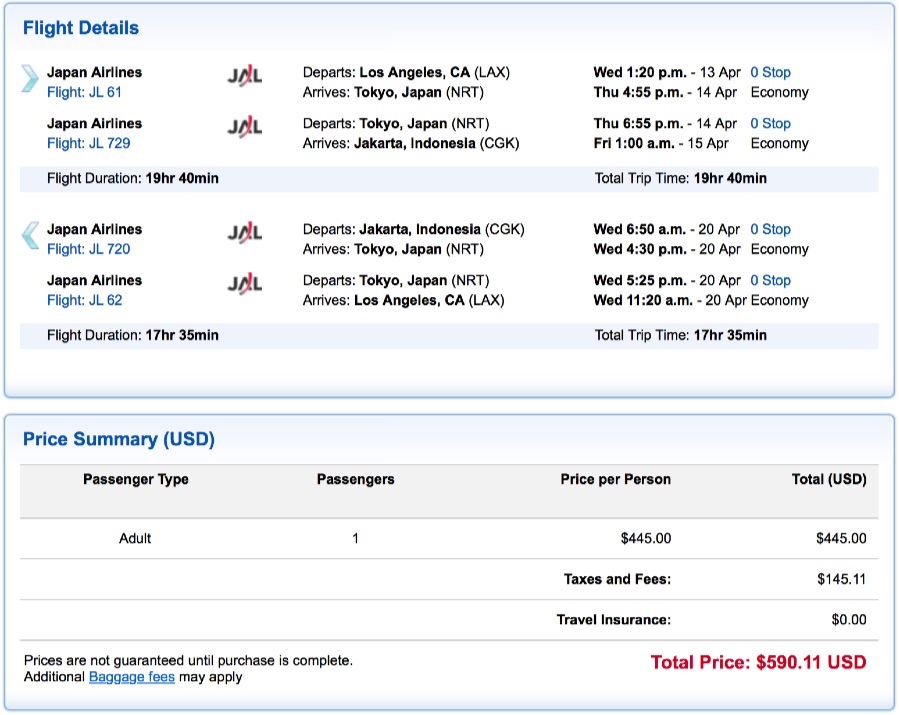Caption: 

The image displays a detailed itinerary for a round-trip journey with Japanese Airlines. The flight departs from Los Angeles (L.A.) on Wednesday at 1:20 PM, traveling non-stop to Tokyo, arriving at 4:55 PM the following day. From Tokyo, the next leg of the journey departs to Jakarta, Indonesia, also non-stop, arriving on Friday at 1:00 AM. The cumulative flight time for this route amounts to 19 hours and 40 minutes.

For the return trip: Departure from Jakarta is scheduled for Wednesday at 6:50 AM, arriving in Tokyo at 4:30 PM, again with no stops and in economy class. The final segment departs from Tokyo at 5:25 PM and lands in L.A. at 11:20 AM on the same day, totaling 17 hours and 35 minutes.

The total time for this travel itinerary is highlighted in darker blue boxes, whereas the financial breakdown is presented underneath. The total price is itemized as $445.00 for one adult passenger with an additional $145.11 for taxes and fees, bringing the total cost to $590.11, clearly indicated in red.